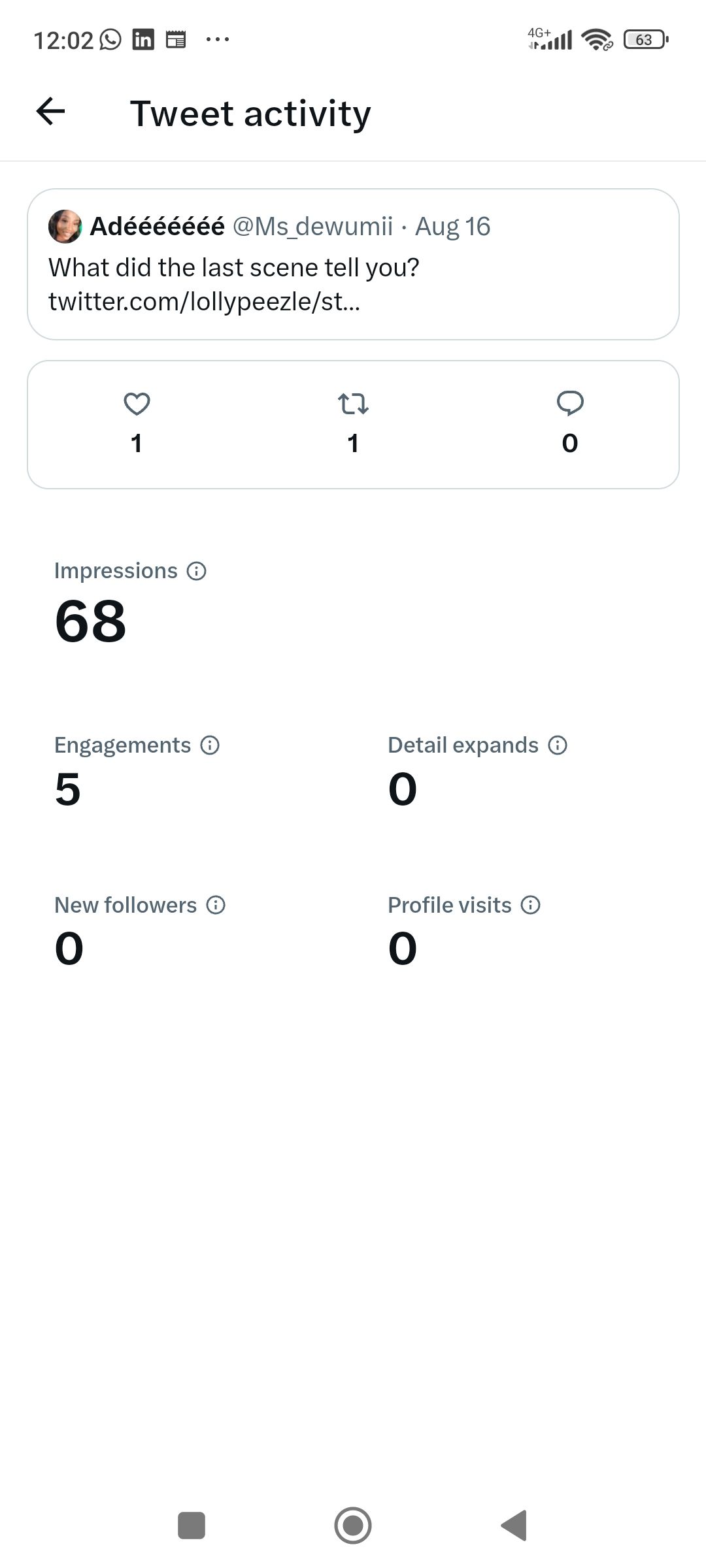This image is a screenshot captured on a cell phone display. In the top left corner, the time is shown as 12:02, while the battery level indicator on the top right reflects a charge of 63%. The page displayed on the screen is titled "Tweet Activity."

The content below this header reveals a user reply stating, "What did the last scene tell you?" This interaction comes from a user named Miss_Underscore_D_Umlee and it was posted on August 16th. The activity metrics indicate the following: one retweet, zero comments, one like, 68 impressions, five engagements, zero new followers, zero profile visits, and zero detail expands.

The background of the page is completely white, with all the text in black. At the very bottom of the image, the standard three navigation buttons of the Android interface are visible.